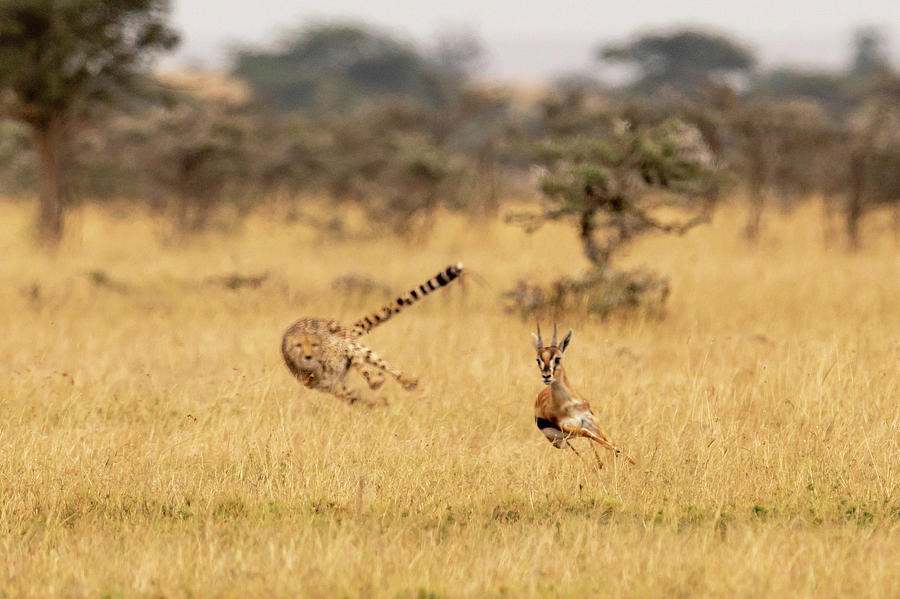In this striking image taken in the wild, a tense moment unfolds in the African plains. The foreground is dominated by a patch of tall, beige-colored grass, through which a baby impala leaps desperately in mid-air. Its delicate frame, adorned with small spiky horns, a brown face, white eye rings, a black stripe down its side, and a white belly, is captured in vivid detail. Behind it, a cheetah, identifiable by its sleek light yellow coat dotted with black spots and a black-striped tail, matches its trajectory, also airborne in a fierce chase. Both animals are in sharp focus, contrasted against a blurred backdrop of dry, olive-leaved trees and a muted gray sky, amplifying the intensity of the predator-prey dynamic. The cheetah's agile form, leaning in a leftward motion with its tail up, highlights its speed and power, while the impala's frantic leap embodies a fight for survival within the vast, open expanse.